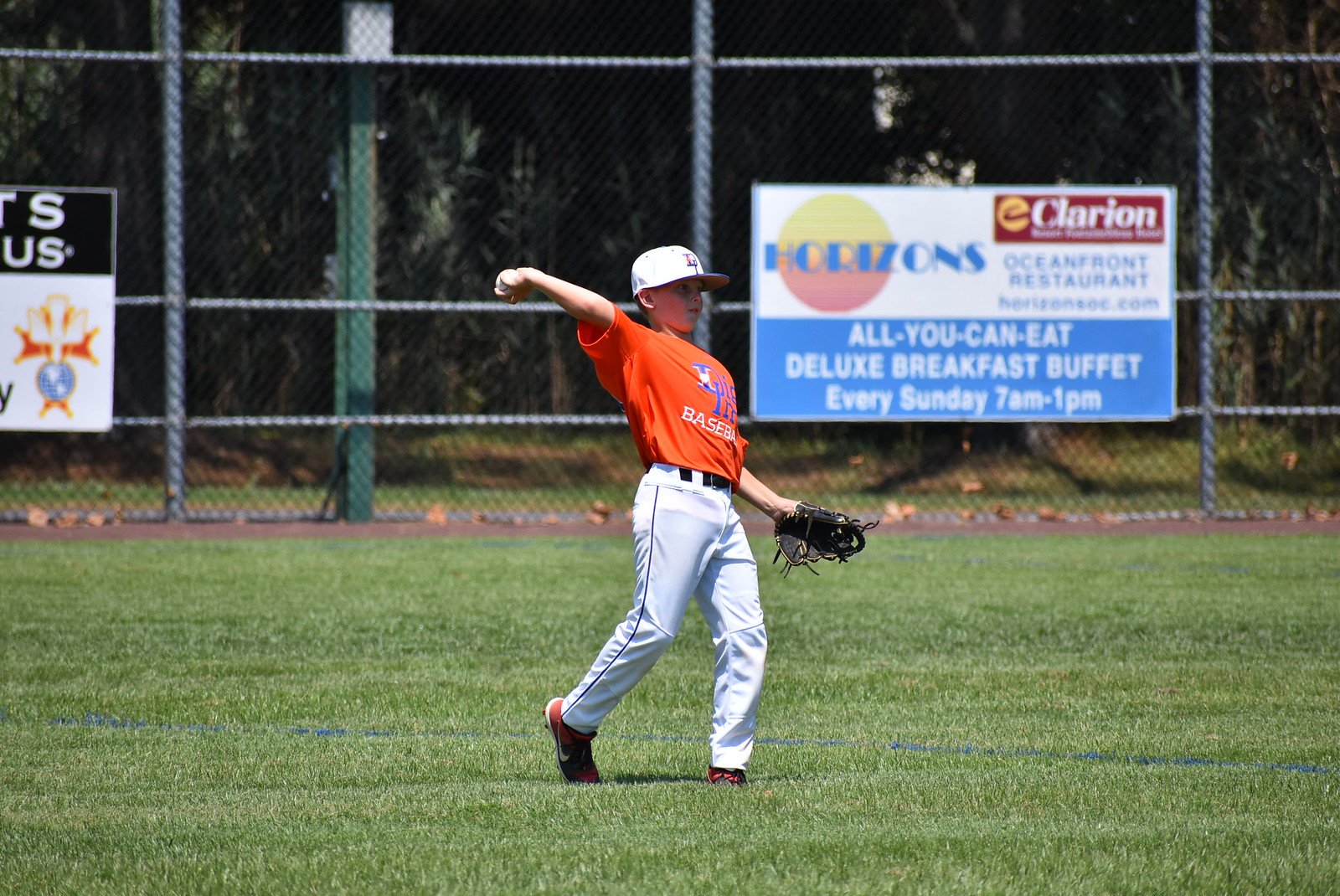The image captures a young boy, likely a Little League player, poised in mid-action as he prepares to throw a baseball. He is positioned in the center of a lush, green outfield enclosed by a chain link fence. The boy is outfitted in a vibrant orange T-shirt adorned with blue and white lettering that spells "baseball," though the full text is partially obscured due to his pitching stance. He also wears white baseball pants and red and black sneakers, with a white cap perched on his head. His right arm is pulled back, ready to release the ball, while his left hand, equipped with a catcher's mitt, hangs down by his side.

In the background, a large advertisement dominates the right side of the fence. The sign features the words "Clarion Horizons" against a backdrop of an orange and yellow ball, along with an offering of an "all-you-can-eat deluxe breakfast buffet every Sunday, 7 AM to 1 PM" displayed in white lettering on a light blue background. To the left side of the image, another billboard partially enters the frame, revealing only fragments of text and symbols. The setting is a fenced-in, grassy field with hints of a wooded area beyond the fence, contributing to the overall vibrant and dynamic atmosphere of the Little League baseball game.